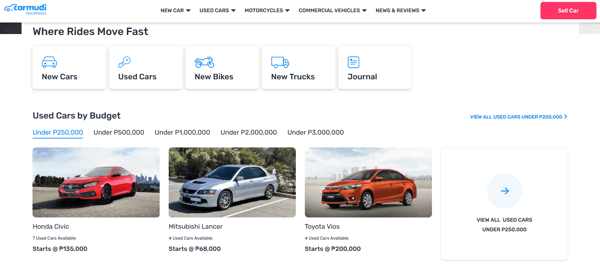**Webpage Screenshot Descriptive Caption**

The image showcases a webpage design set against a clean, all-white backdrop. In the upper left-hand corner, a blue logo features the outline of a car trunk pointing to the left, viewed in profile. To the right of this logo, the brand name "CARMUDI" is prominently displayed in blue capital letters. Below the brand name, another line of blue text appears, although it is rendered blurry and unreadable.

Centrally positioned at the top of the page, various categories of vehicles are labeled in black text with drop-down arrows beside each. The categories include "New Car," "Used Cars," "Motorcycles," "Commercial Vehicles," and a final category that seems to say "Views & Reviews," also with a drop-down arrow. 

In the upper right-hand corner, there is a red bar that reads "C-CAR" in white text. Beneath this bar, on the left side of the page, a slogan reads "Where rides move fast" in black text. Below this slogan, a series of five consecutive white boxes depict different categories of vehicles and content. Each box features a blue icon at the top left and associated category names beneath:

1. A blue car icon with the label "New Cars"
2. A blue key icon labeled "Used Cars"
3. A blue motorcycle icon labeled "New Bikes"
4. A blue moving van icon labeled "New Trucks"
5. A blue paper icon labeled "Journal"

Underneath these boxes, a black heading states "Used Cars by Budget," followed by budget categories expressed in blue and black text:

- 'Under P250,000' (in blue, underlined)
- 'Under P500,000' (in black)
- 'Under P1,000,000' (in black)
- 'Under P2,000,000' (in black)
- 'Under P3,000,000' (in black)

Adjacent to this section, on the right-hand side of the page, a blue text link reads "View all used cars under P250,000."

Below these sections are three pictures of cars:

1. A red two-door sedan labeled "Honda Civic" with a price starting at P135,000.
2. A gray four-door car labeled "Mitsubishi Lancer," starting at P68,000.
3. An orange four-door car labeled "Toyota Vios," starting at P200,000.

To the right of these images, there is a small white box featuring a gray circle with a blue left-pointing arrow at the top. Beneath this symbol, the text "View all used cars under P250,000" is written in black.